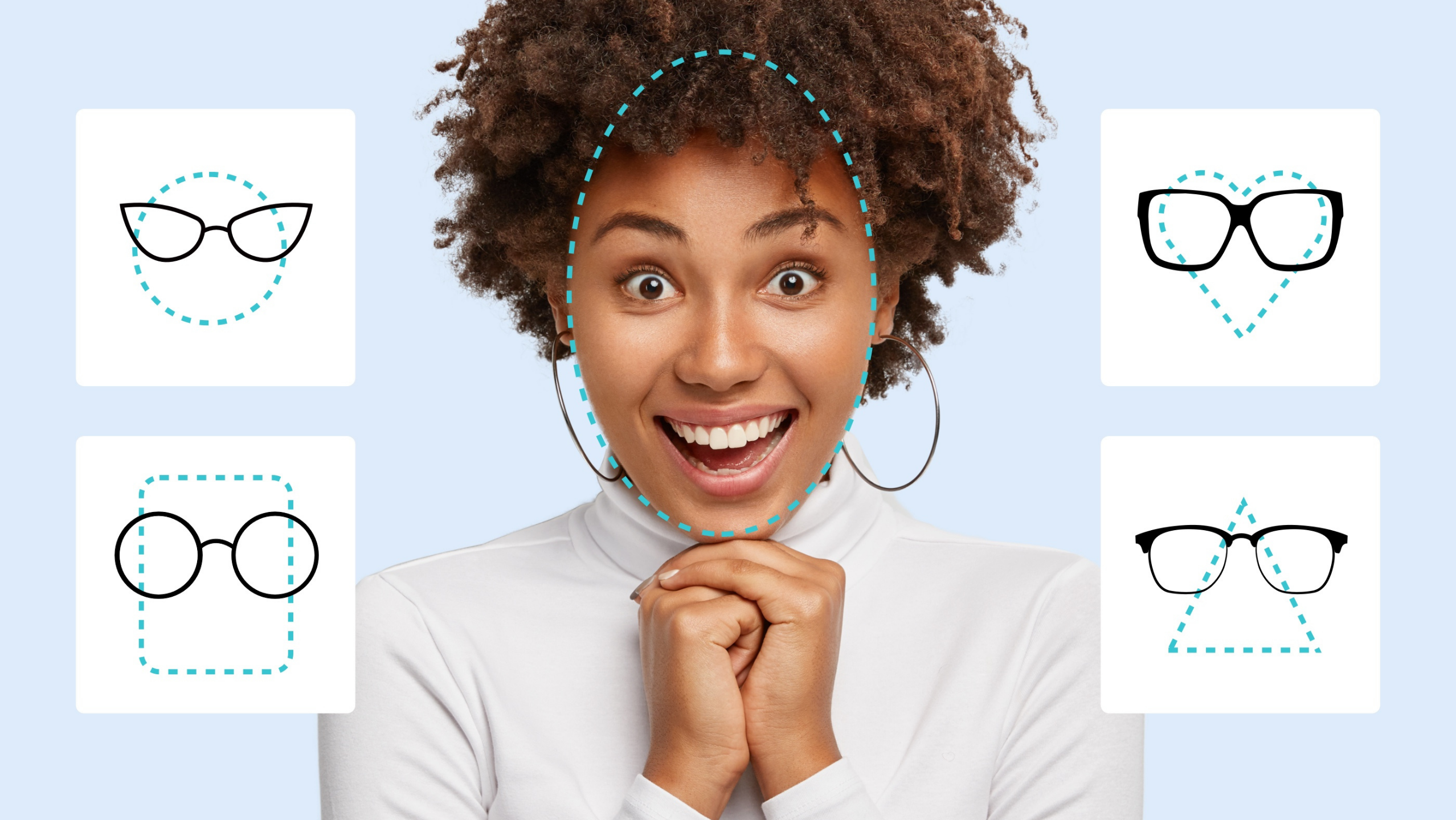This image features a happy Black woman smiling directly at the camera. She has short to medium-length hair, is wearing large round hoop earrings, and a thin white sweater. Around her face, there's a dotted line indicating her face shape. The background is a soft baby blue color. Flanking her are four white squares, two on each side, each containing illustrations of different face shapes paired with suitable glasses. The top left square shows a circular face with cat-eye glasses; the bottom left features a rectangular face with Harry Potter-style round glasses. On the right, the top square displays a heart-shaped face with large glasses, and the bottom square depicts a triangle-shaped face with distinct eyebrow line glasses. This setup is reminiscent of promotional photos often seen in doctor's offices or eyeglass shops, guiding customers on the best glasses for their face shape.